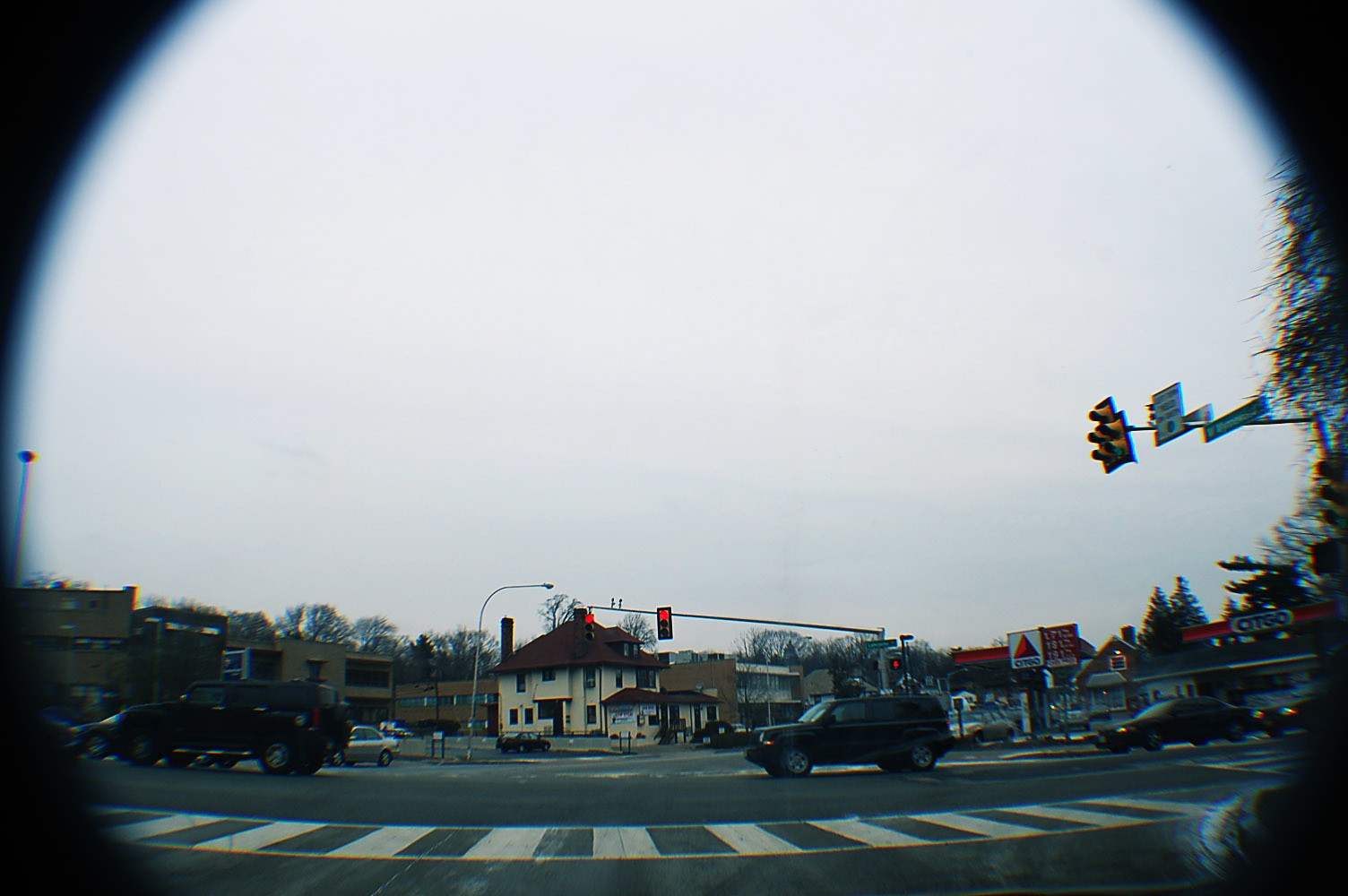Through the lens of what appears to be a telescope or a circular frame, the image captures a bustling urban intersection from an elevated perspective. The main focal point is a brightly illuminated pedestrian crosswalk, with the surrounding scene gradually fading into darkness around the edges, adding a vignette effect. In the middle ground, several cars are seen traversing the intersection, while a glaring red traffic light holds their attention, signaling them to stop. Directly across the street, a prominent white building topped with a brown roof stands out. Adjacent to it is a Sitco gas station, its signage and facilities partially in view, though the gas prices remain indiscernible. Beyond this primary scene, a collection of smaller structures populates the background—one appearing to be a parking lot, while others resemble modest office buildings, contributing to the urban tapestry. The perspective hints at the photo being taken from within a vehicle, adding a layer of narrative to the urban tableau.